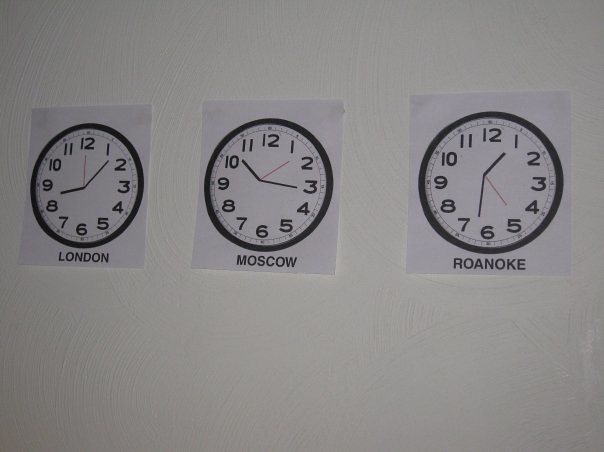The image depicts three white pieces of paper taped onto a light gray wall, each featuring a printout of a clock face representing different time zones. The clocks are simple with a black rim, bold Arabic numerals, a minute and an hour hand, and a red second hand on a white face. The first clock, labeled "London," shows the time as approximately 8:05 or 8:06. The second clock, labeled "Moscow," displays the time as 10:15. The third clock, labeled "Roanoke," shows the time as about 1:32 or 1:34. The pieces of paper appear to be taped to the wall with small balls of Scotch tape.